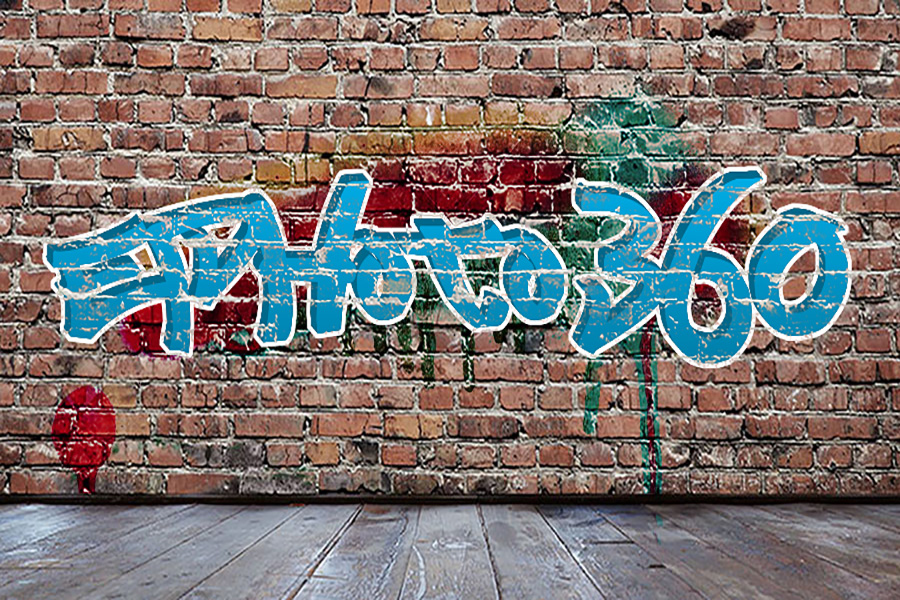This color photograph captures an interior scene with a prominently graffiti-tagged brick wall. The bricks are a reddish-brown hue, typical of traditional brickwork. The floor in front of the wall is composed of gray wooden planks, enhancing the indoor setting. The graffiti appears to spell out "E-photo 360," although the stylized blue letters with white outlines make the first couple of letters slightly ambiguous. Accentuating the graffiti, there are splashes of red and drippings of green paint, adding to the wall's vibrant, artistic chaos. Notably, there's a distinct red splotch in the lower-left corner of the wall. The overall effect is a visually striking combination of urban street art within a presumably indoor space.